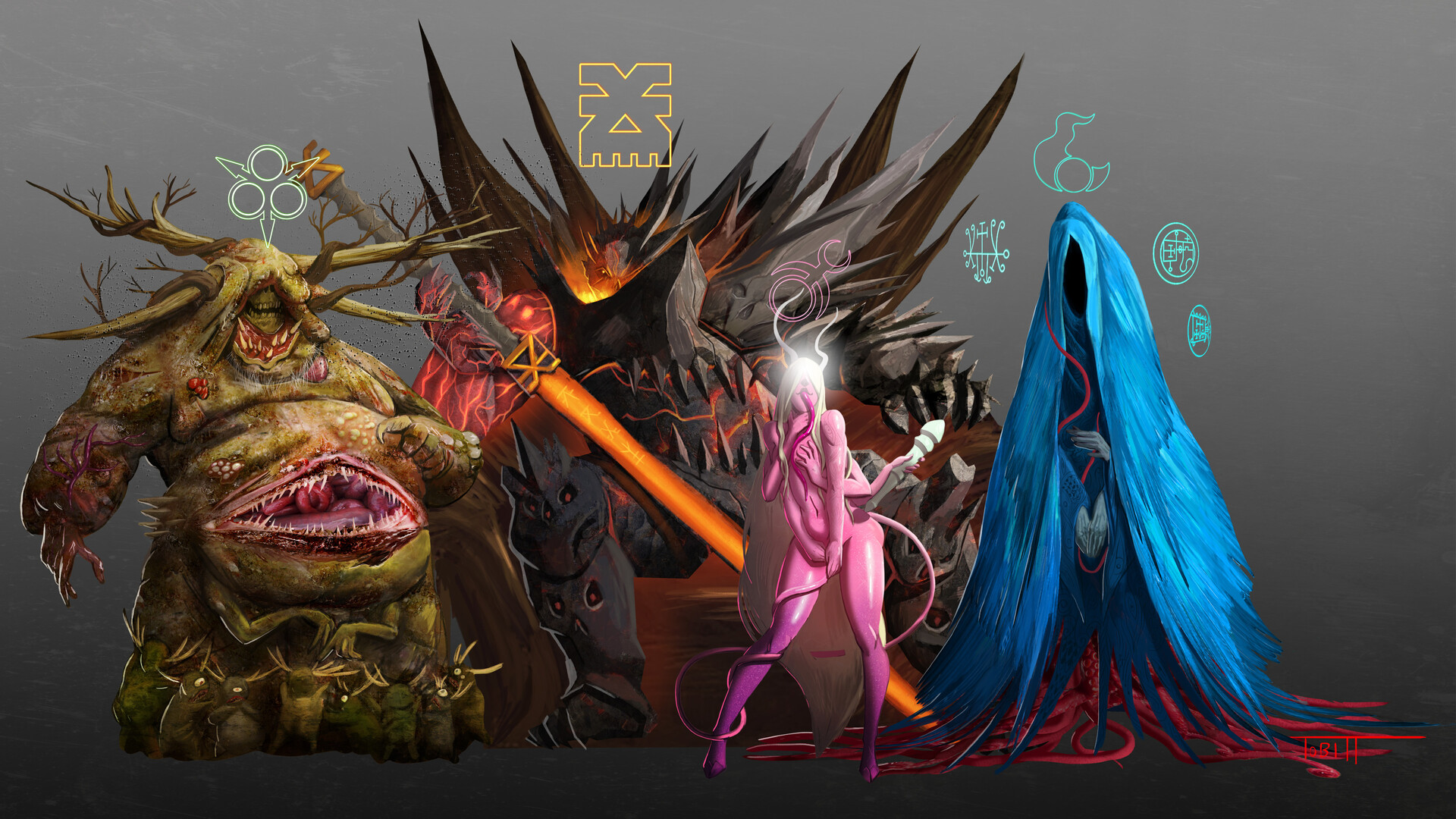This image is a horizontally oriented, digitally animated character sheet set against a dark gray, smoky background. It features four distinct, fantasy horror creatures lined up from left to right. On the left, there's a large, obese green monster with tree branches protruding from its head and a gaping mouth in its stomach, accompanied by a symbol above its head. In the background, next to the green monster, is a rock and lava creature wielding a red sword, with black spikes emerging from its body. Centrally placed in the foreground is a pink, somewhat sexualized fairy-like devil with white hair, multiple hands, and a tail, which stands out with its vines or tendrils wrapping around its leg. On the far right, there's a tall, ghostly blue figure with an obscured face and three hands, giving it a mysterious, ink-like appearance. Each character has distinct symbols above their heads, enhancing the mystical aura of the composition. The animation is noted for its smooth and detailed digital artistry, contributing to the overall eerie and fantastical atmosphere.